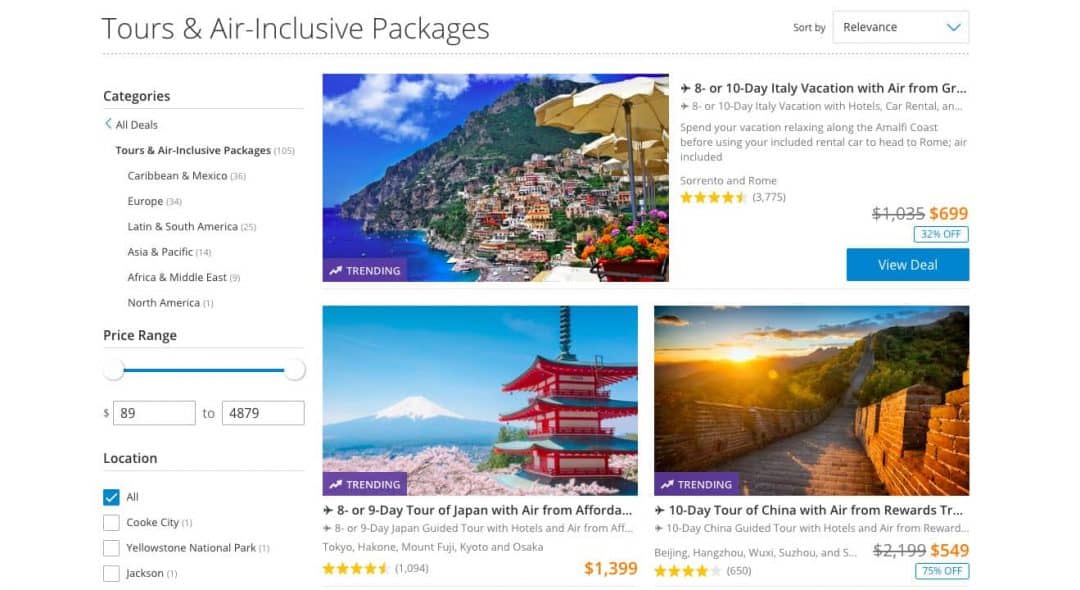Here's the cleaned-up caption:

---

The image captures a webpage titled "Tours and Air Inclusive Packages" displayed on a computer screen. Centrally, the page features three highlighted vacation packages with accompanying descriptions. The first image showcases a picturesque, sunny town nestled on a mountainside overlooking the ocean, featuring a yellow umbrella and vibrant flowers in the foreground. The description promotes an 8 or 10-day Italy vacation with air travel from GR, highlighting Sorrento and Rome. This package has received a 4.5-star rating from 3,775 reviewers. Original pricing of $1,035 has been discounted to $699, marked in orange, with a blue box indicating 32% off. Below, a larger blue rectangle with white text reads "View Deal."

Additionally, the page includes images and descriptions for vacations in the Tokyo and Beijing areas. 

On the left side, a vertical menu lists various categories, with "Tours and Air Inclusive Packages" highlighted, reflecting the current selection. Other categories include Caribbean and Mexico, Europe, Latin and South America, etc. Users can filter options by price range and locations, with a checkbox for "All" prominently marked in blue.